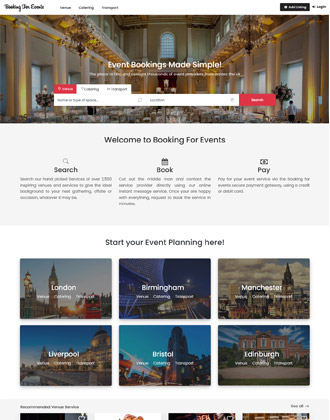The image depicts a low-resolution website with poor readability. The webpage features a white background, with a prominent black button located on the right side of the screen. At the top, there is a navigation bar; however, the text is illegible. 

Beneath the navigation bar, there is a wide photo stretching across the screen that bears the slogan, "Event Bookings Made Simple." Overlaying this photograph is a bar with a red button beside three tabs; the red button's text is unreadable, and one tab is highlighted in red while the other two are white.

Further down, the site contains a banner reading, "Welcome to Booking for Events, Search Book Pay." Below this heading, there are two rows with three images each, showcasing various cities including London, Birmingham, Manchester, Liverpool, Bristol, and Edinburgh. Text is overlaid on these images, but it is too small to decipher.

The color scheme throughout the site includes a diverse palette with blue, brown, red, gray, black, white, gold, green, dark brown, light brown, and orange. Despite the vibrant colors, the overall design suffers from low resolution, making detailed viewing difficult.